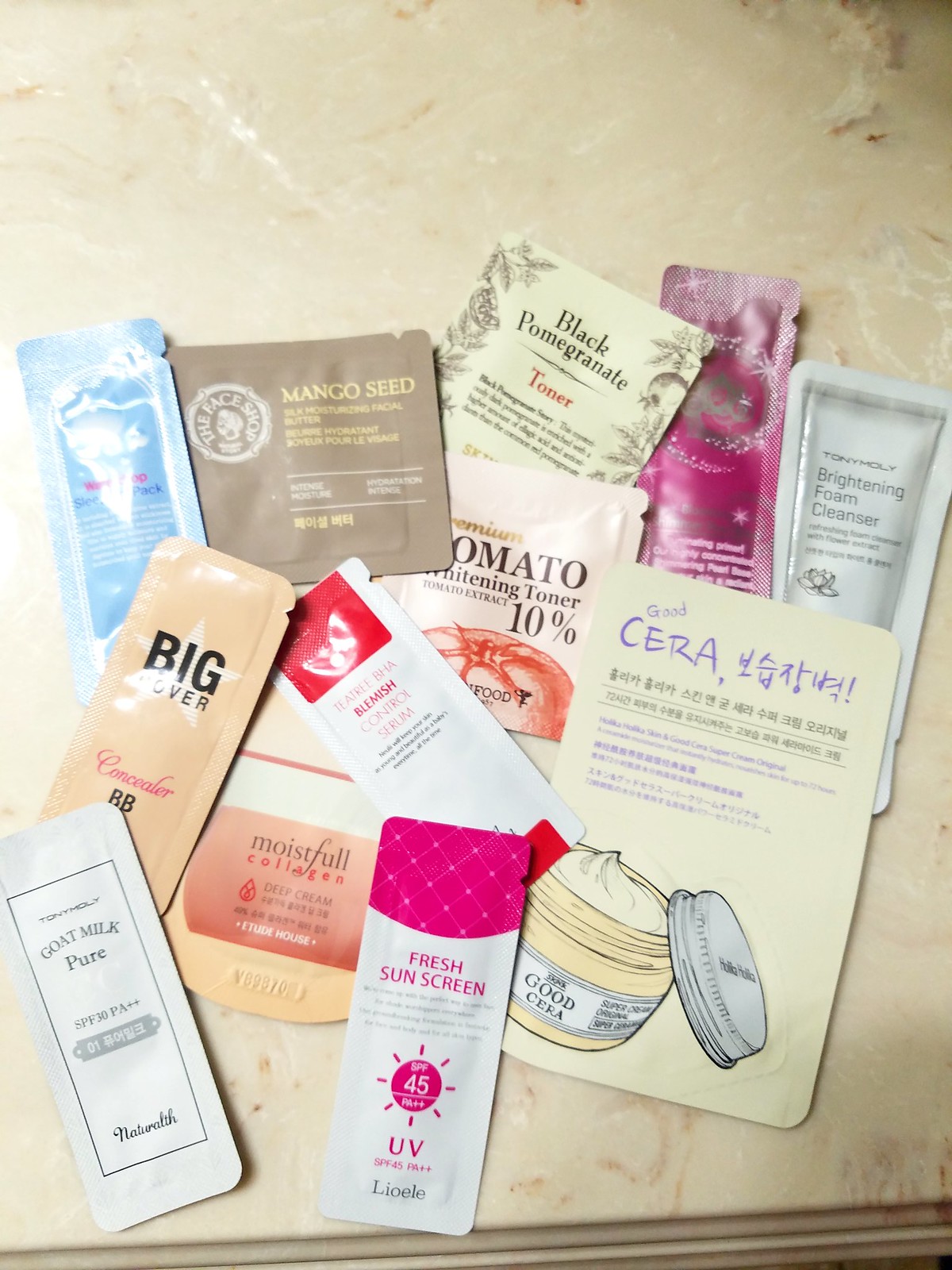This image showcases an assortment of 12 sample packets of beauty products carefully arranged on a stunning marble countertop. The countertop features a luxurious beige base with striking brown and white undertones and is finished with a decorative edge along the bottom, where a subtle strip of brown is visible.

Starting from the left, the first sample packet is a vibrant blue with white lettering, although the text is obscured by light reflection. It rests atop another packet, brown in color, bearing a logo resembling a woman encircled by text, with "Mango Seed" prominently displayed in yellow letters.

Moving to the right, the next packet is a light yellow sample labeled "Black Pomegranate Toner," adorned with floral or botanical designs along the edge. Partially tucked beneath it is a vivid purple and bright pink packet featuring a swirl of white bubbles, but the lettering is indiscernible due to the light reflection.

The last packet in this row is a greenish packet marked "Brightening Foam Cleaner." Following this, a beige packet with the word "BIG" is visible; next to it, a pink packet reads "Moistful." Further along, a red and white packet's text is unreadable, followed by a light yellow one that states "Something Sarah." A white packet identifies itself as "Goat Milk Pure," and finally, another pink and white packet is labeled "Fresh Sunscreen."